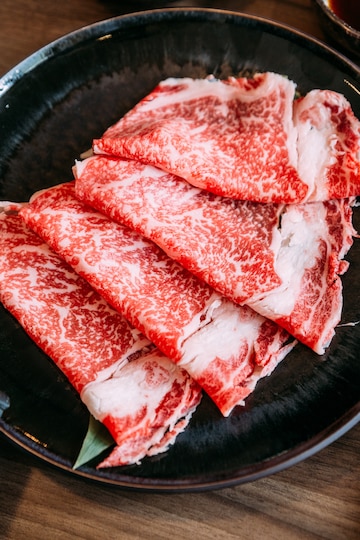The image depicts a vertical, rectangular photo of a black, round plate, placed on a darker wooden table with visible grains running through it. In the center of the plate, there are four very thinly sliced pieces of raw Wagyu beef chuck. Each slice has been intricately folded once in half and layered partially on top of one another, allowing visibility of each piece's marbled red and white texture. The meat displays a thick white strip of fat running horizontally along the edges, emphasizing its rich, uncooked quality. A small lettuce leaf peeks out from beneath the meat, adding a touch of greenery. In the upper right corner of the image, another piece of pottery is partially visible, though its exact nature remains unclear. Overall, the presentation highlights the intricate details of the beef's marbling against the contrasting dark plate and wooden background.